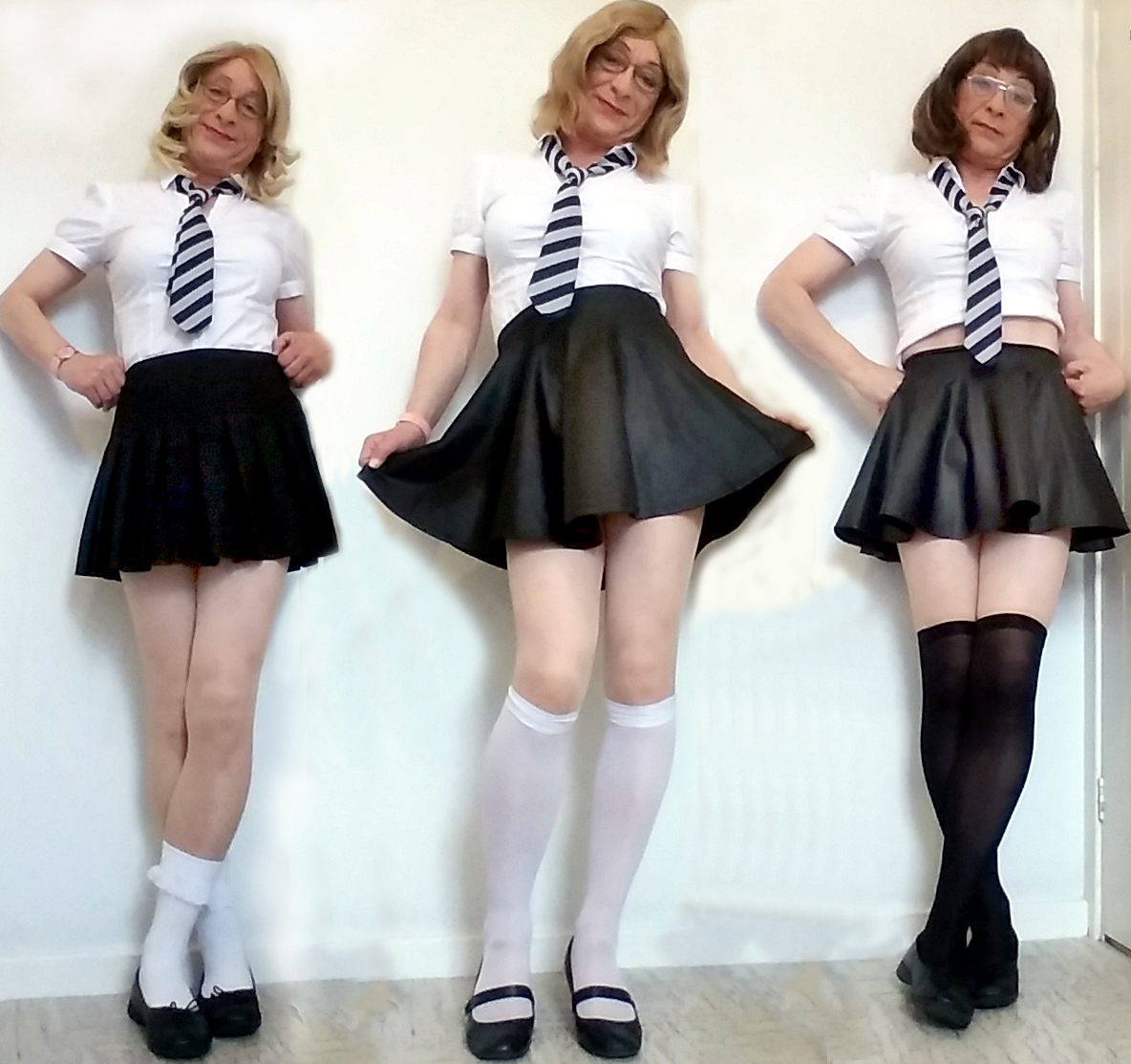This detailed color photo features three individuals standing against a white wall with a baseboard, positioned on a floor that is a mix of light gray and tan with splotches of tan. Each person is dressed in a distinct schoolgirl costume, giving the impression that they might be the same individual photoshopped into the image three times, yet they could also be separate people.

The individuals are adorned with short white midriff-bearing T-shirts and blue and gray striped neckties with alternating black and dark gray stripes. Their skirts, all short and pleated, showcase different materials: the one on the left wears a standard cotton skirt, the one in the middle sports a silk-like skirt, and the one on the right displays a ruffled leather skirt.

Additionally, each person dons different types of stockings and footwear. The person on the left has short white socks paired with black dress shoes. The individual in the middle wears knee-high, slightly see-through white stockings with black sandals. The one on the right features high black fishnet stockings extending above the knees, complemented by black shoes.

Their headwear includes wigs: the person on the right has a short brunette wig with bangs, while the other two wear short wavy blonde wigs. This image highlights a playful and coordinated sense of style, emphasizing subtle differences in their attire and posing against the minimalist backdrop.